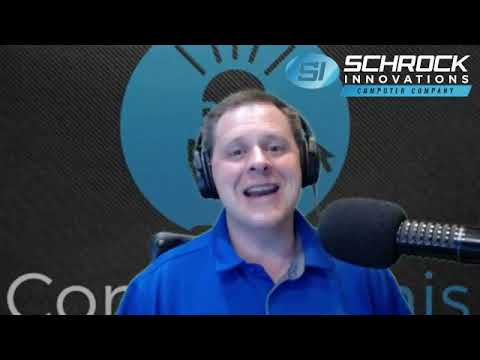The image is a screen grab from a webcam featuring a man mid-speech, seemingly expressive and slightly laughing. He has short brown hair and is wearing a vibrant royal blue polo shirt along with a set of large, black headphones covering his ears. He speaks into a microphone that has a black tip and a silverish-black stand. The background behind him has a gradient, textured charcoal black surface with a partially obscured brand logo and graphical elements, including a blue disc partially visible behind him. The disc has an indistinct microphone symbol, mostly covered by the man. In the upper right corner of the image, white text reads "Schrock Innovations Computer Company" with "SI" placed beside it within a blue oval. The foreground also features a black top and bottom header bar, each about half an inch thick.